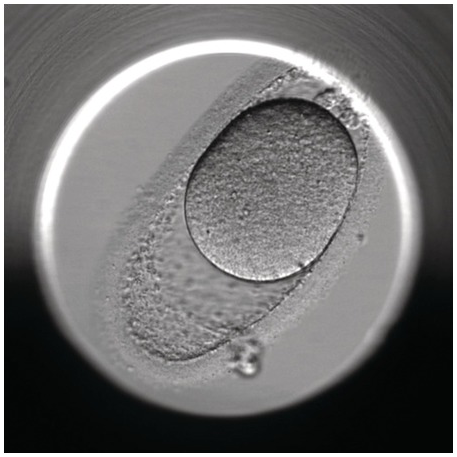This image is a highly detailed, close-up photograph capturing what appears to be the intricate components of a metal lock or machine part, with a visible circular keyhole surrounded by a rough-textured oblong oval shape. The entirety of the foreground features smooth gray metal with subtle circular scratching patterns, reflecting a manufactured, industrial look, likely made of heavy metal or steel. In the background, out-of-focus elements contribute to this metallic landscape, invoking a surreal sense of outer space. The overall appearance is somewhat grainy, adding to the impression of viewing the object through a microscope or a tubular lens, bringing out the fine edges and rough interior details that suggest layers within layers, evoking an almost cellular structure.